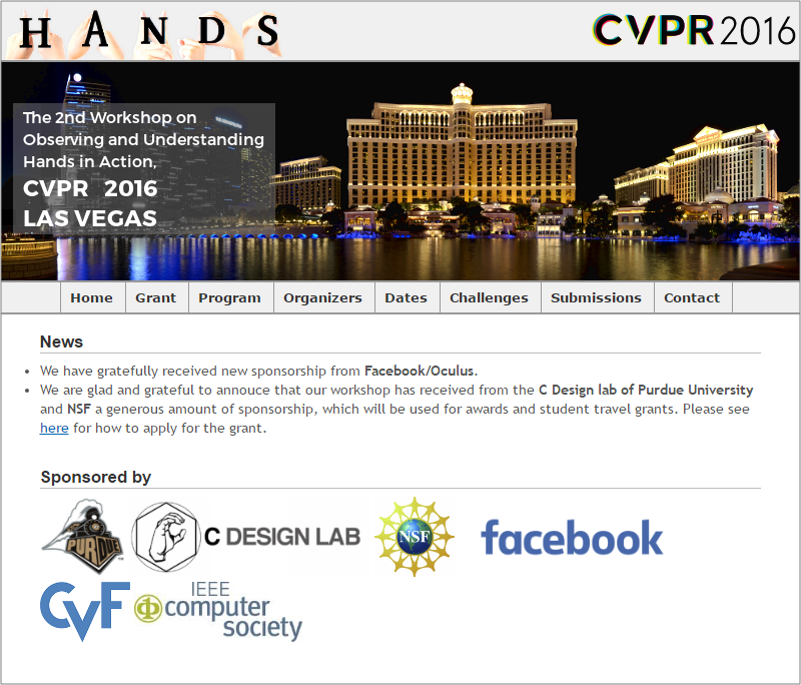This image appears to be from a website dedicated to hand research or hand recognition technology. In the upper left-hand corner, the word "HANDS" is displayed with each letter spaced apart significantly, almost double-spaced. Behind each letter, there are hands forming various symbols: two hands behind the "H" have index fingers pointing outward, creating a visual effect, while the "A" is formed by two hands positioned together to resemble the letter "A". 

In the upper right-hand corner, the text "CVPR 2016" is clearly visible. Below this, a panoramic banner stretches across the width of the image, showcasing an evening cityscape scene with multiple buildings illuminated against the night sky. In the foreground, a body of water reflects the lights from the buildings. 

To the left of the banner, there is a caption that reads: "The Second Workshop on Observing and Understanding Hands in Action. CVPR 2016, Las Vegas."